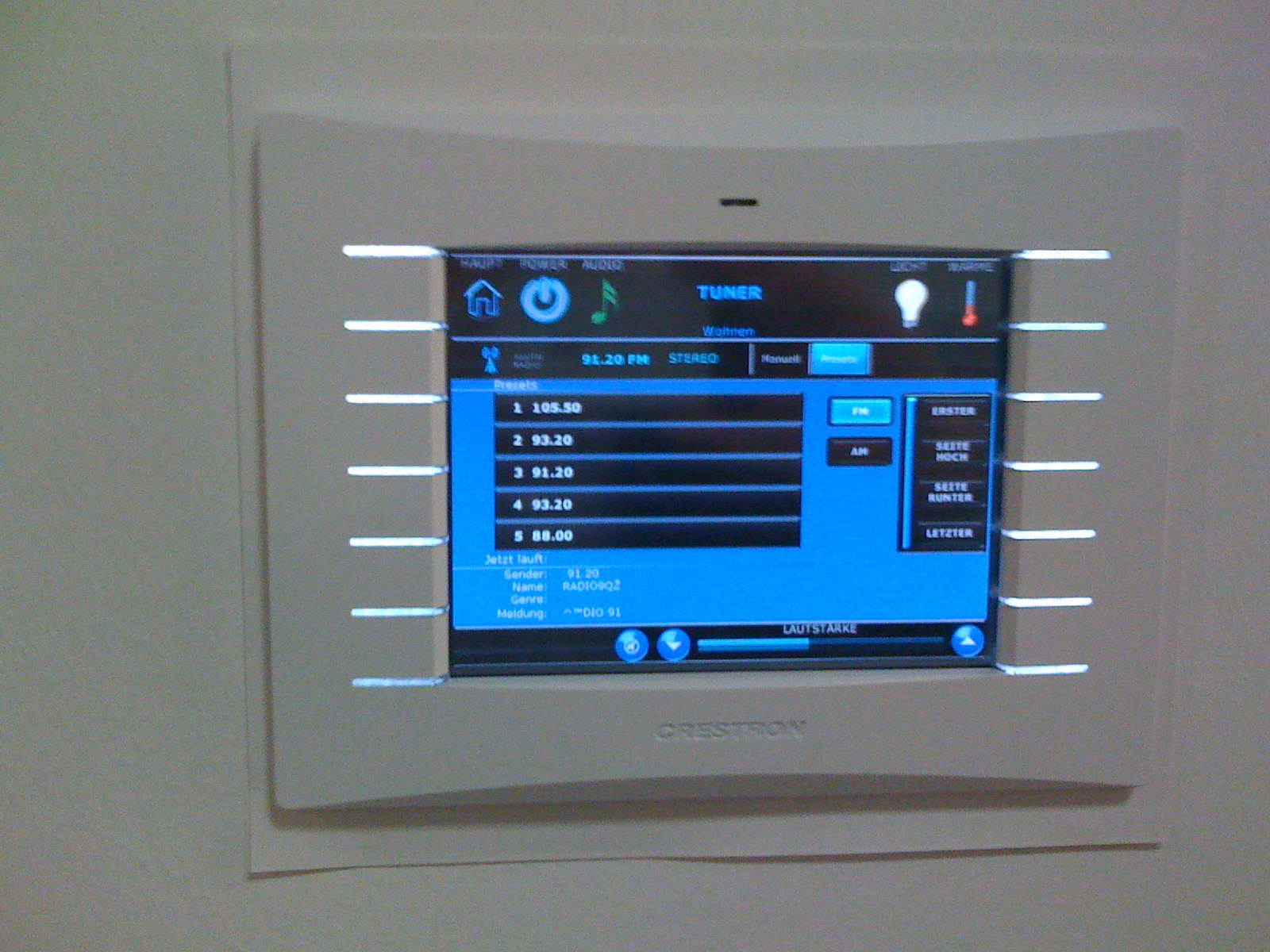This close-up photograph showcases a sleek, modern digital control panel mounted on a pristine white wall. The device itself has a white plastic casing that slightly protrudes from the wall, creating a clean and minimalist look. Centrally, there is a raised rectangular section with gently curved top and bottom edges, enhancing its aesthetic appeal.

Etched at the bottom of this raised section is the brand name "Crestron," indicating the manufacturer's identity. Flanking this central rectangle are two bright horizontal bar lights — one on each side — casting a luminous white glow.

The centerpiece of this device is its screen, which is divided into distinct sections. The top and bottom of the screen feature black bars. Within the top black bar are several symbols arranged from left to right: a house symbol, a power button symbol, an eighth note music symbol, a light bulb symbol, and a thermometer symbol with a red gradient at the bottom. These icons are labeled in small text: "Home," "Power," "Audio," "Light," and "Warmth."

Between the black bars is a blue section that functions as the main display area. It is headed by the label "Tuner" and is categorized under "Presets." The presets are listed as follows:
1. 105.50 
2. 93.20 
3. 91.20 
4. 93.20 
5. 88.00 

Each station is displayed in a black bar with white text, offering a clear and organized view. Overall, this detailed layout exemplifies a high-tech, user-friendly interface designed for seamless home automation control.